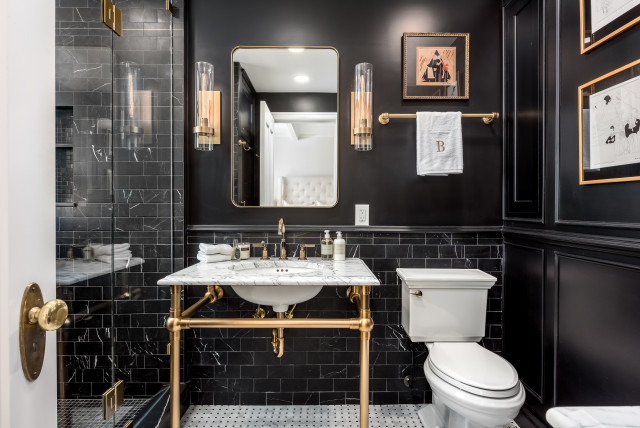The image depicts a stylish and elegant bathroom interior with predominantly dark grey walls adorned with grey trim and black marble subway tiles on the lower half. A white toilet is positioned on the bottom right, while to the center-left stands a striking gold pedestal sink with a white Carrara marble basin, golden faucet fixtures, and a washcloth. The sink is complemented by a cabinet mirror framed in gold, flanked by gold sconces. The floor is crafted from white Carrara marble, adding a touch of sophistication. On the left, a glass-walled shower showcases the same black marble subway tile as the walls. The door, partially visible on the left side, features a gold handle and doorknob. Hanging above the toilet is a gold towel bar with a hand towel adorned with a gold bead, and a framed piece of artwork. Additional framed pictures are mounted on the right-hand side of the wall, contributing to the decorative aesthetic. The combination of gold accents, marble surfaces, and framed artwork reflects a luxurious and thoughtfully designed space.